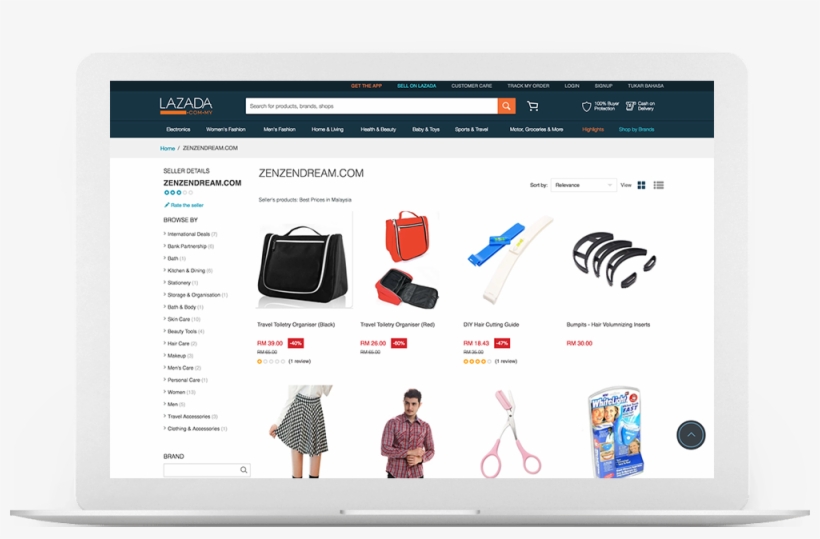The image is a screenshot from the website LASDA, showcasing its user interface with various key elements. At the top, prominently displayed is the website's name. Beneath it, a search box allows users to explore the site’s offerings. Adjacent to the search box is a shopping cart icon for easy access to selected items. Following these, two icons likely serving functional purposes such as user account and support, are positioned. Below this section, several navigation tabs categorize the site's content into directories including Women's Fashion, Men's Fashion, Home and Living, Health and Beauty, and Toys, Sports, and Travel.

Further down, the image highlights the domain name Zenzendream.com twice, suggesting a specific branding or affiliate linkage. Dividing the page, four product showcase sections are prominently displayed, both at the top and bottom of the page, collectively featuring a variety of different products available for purchase. These elements together create an organized and user-friendly layout facilitating easy navigation and shopping experiences on LASDA. The URL Zenzendream.com appears prominently, hinting that it might be the featured brand or a focused section within the LASDA site.